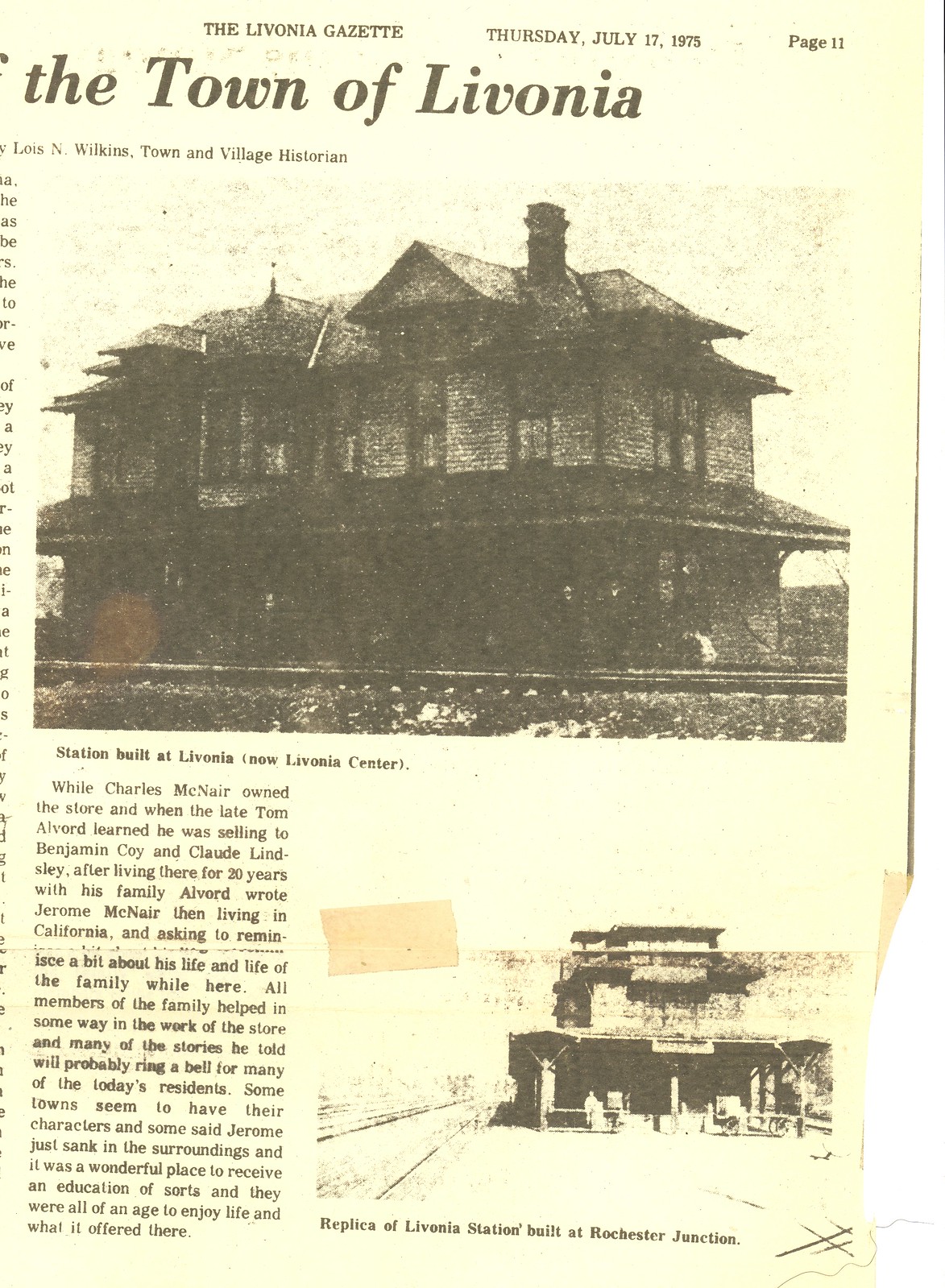This image is a digital screenshot of a yellowed, torn-out newspaper clipping from the Livonia Gazette, dated Thursday, July 17, 1975, page 11. The visible portion of the clipping includes the right-hand side. At the top of the page is an image captioned with "Replica of Livonia station built at Rochester Junction," depicting a large, two-story train station with train tracks running alongside its length. Below this is a smaller image showing the train station from a different angle. The larger image caption suggests that the structure is a significant representation of the local train station. Adjacent to the smaller image, there is a partially visible, detailed paragraph elucidating the history and context of the Livonia station, mentioning notable individuals such as Charles McNair and Tom Alvord and their contributions to the town, indicating the station's long-standing impact on the community's development and daily life.